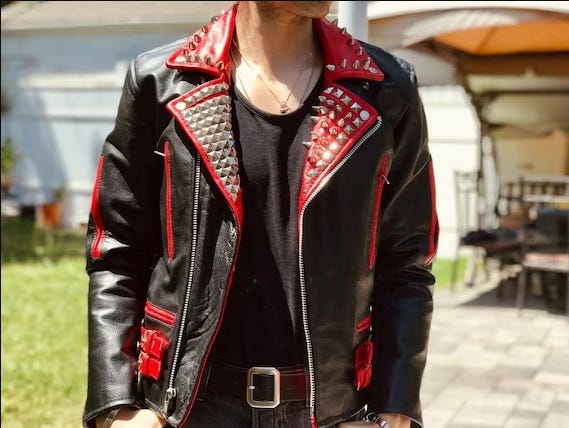In this high-quality image, we observe a close-up of a human torso, cropped from the chin to just below the waist. The person, who has scruff on their chin and Caucasian skin, stands outside near a house with the indistinct background showing grass to the left and a patio to the right. The patio features a swing with a covered umbrella and a table with chairs. The individual is adorned in a bold, punk-inspired ensemble comprising a black and red jacket. The jacket is predominantly black with red accents lining the interior, collar, and zippers. Silver studs and spikes embellish the collar and front area, amplifying the punk aesthetic. Additional details include orange leather pockets under the arms and zippers on the sleeves. Beneath the jacket, the person wears a black t-shirt and two small gold necklaces. Their waist is cinched with a large brown belt featuring a substantial silver buckle, and they appear to be wearing dark jeans with their hands casually inserted into the front pockets.